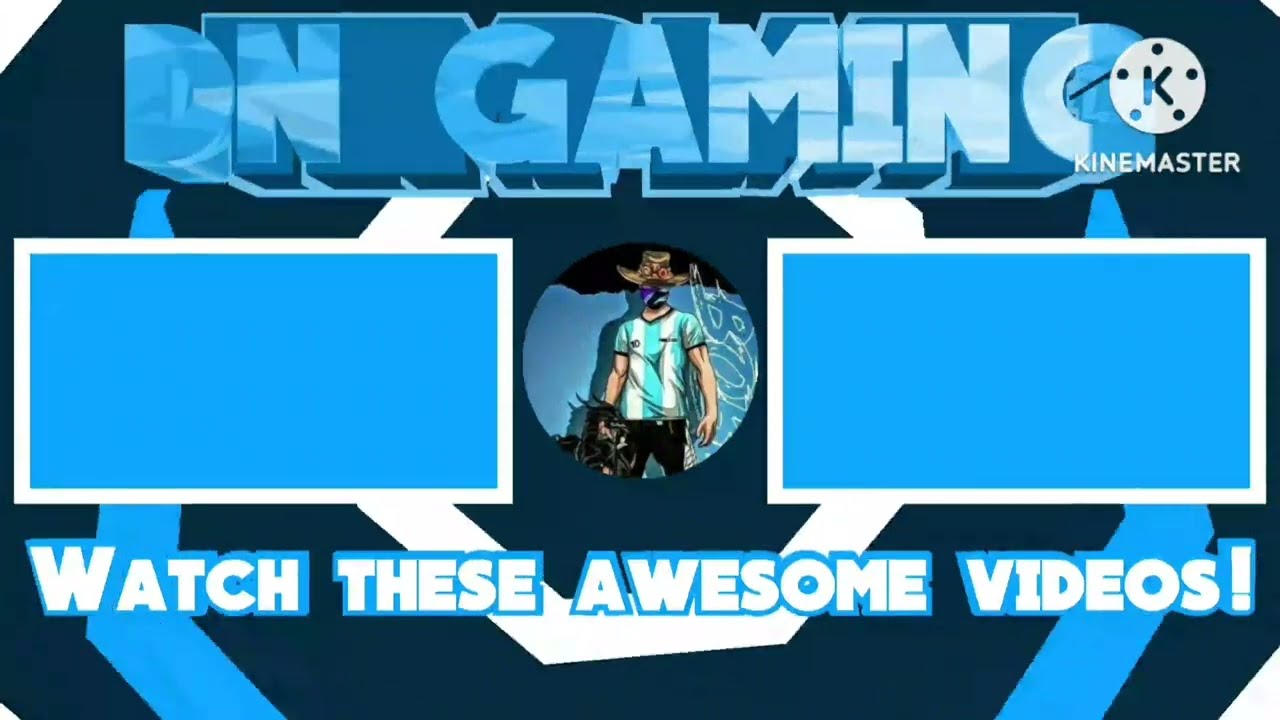The banner features a deep dark greenish-blue background with prominent, thick, 3D block letters across the top that spell out "DNGaming" in uppercase blue letters with a shadow effect. Under the "G" in "Gaming," there is a white circle containing a "K" in the center, accompanied by five smaller holes around its edge and the text "KineMaster" beneath it. In the center of the banner, there's a circular graphic of a man wearing a vertically striped shirt in black and white, black pants, a wide straw hat, and a black mask. He is holding a black item in one hand, with his other hand hanging by his hip. Flanking him on either side are blue squares outlined in white. At the very bottom, the phrase "WATCH THESE AWESOME VIDEOS" is displayed in uppercase white letters with a blue outline, where "WATCH" is larger than the rest of the text.